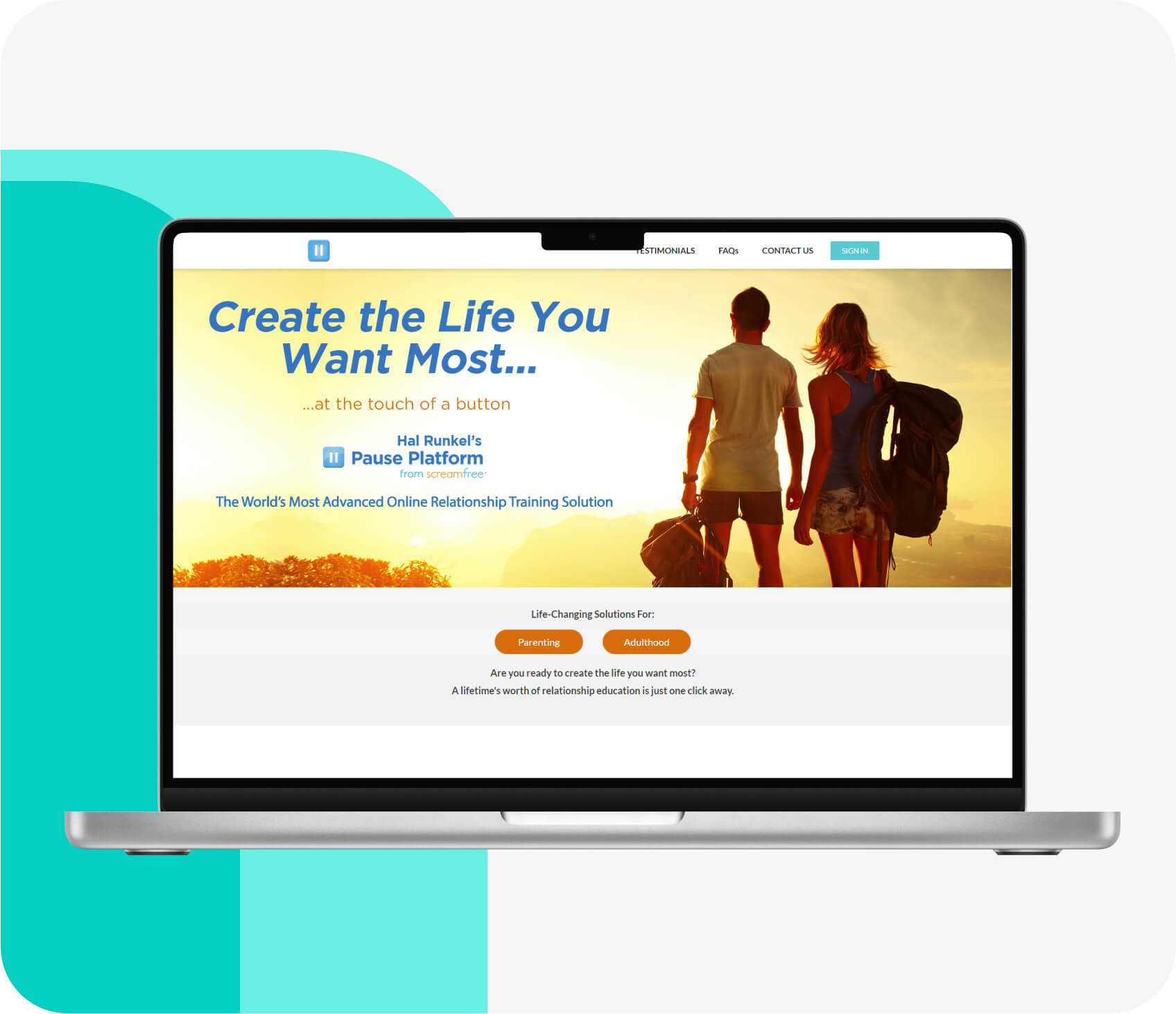The image is a vibrant color photograph featuring a computer monitor set against a white and mint green background. Displayed on the monitor is an inspiring message overlaid on a breathtaking photo of a yellow sunset that reads, "Create the life you want most at the touch of a button. Hal Runkle's Pause Platform from Scream Free, the world's most advanced online relationship training solution." In the foreground of the sunset image, two individuals stand with their backs towards us, gazing out at the serene sunset. Below the monitor's display, a white footer spans the width of the image, showcasing centered black text stating, "Life changing solutions for." The footer also includes two orange buttons placed side by side—one labeled "Parenting" and the other "Adulthood." The caption below reads, "Are you ready to create the life you want most? A lifetime's worth of relationship education is just one click away."